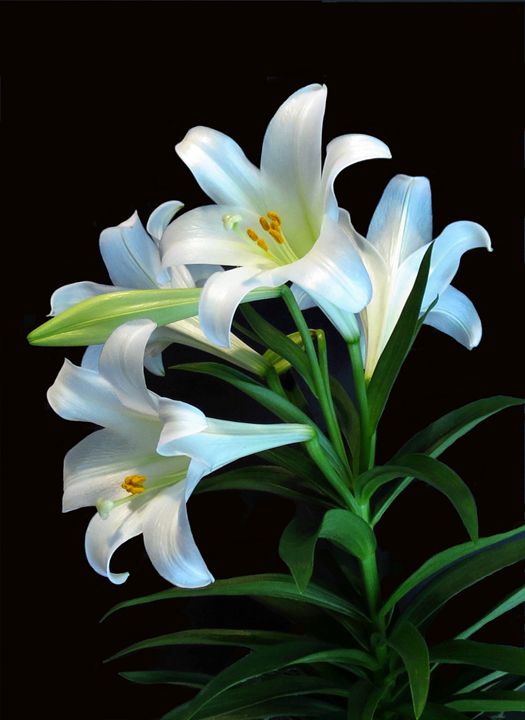This image showcases a professional, striking photograph of Easter lilies set against a black background. The main subject is a single central stalk, adorned with numerous green leaves that gracefully extend outward. The stalk culminates in a cluster of blooms, with four fully opened white flowers and one yet-to-bloom green bud. Each open lily flower is shaped like a wide funnel, featuring six pointed petals that elegantly flare outwards. Inside the flowers, vibrant orange-tipped stamens add a contrasting splash of color. The black backdrop enhances the purity of the white petals and the vividness of the green leaves, making the overall presentation particularly striking. This meticulous depiction of the Easter lilies, likely intended for a product page, highlights the beauty and intricacy of the flowers in a detailed and visually appealing manner.